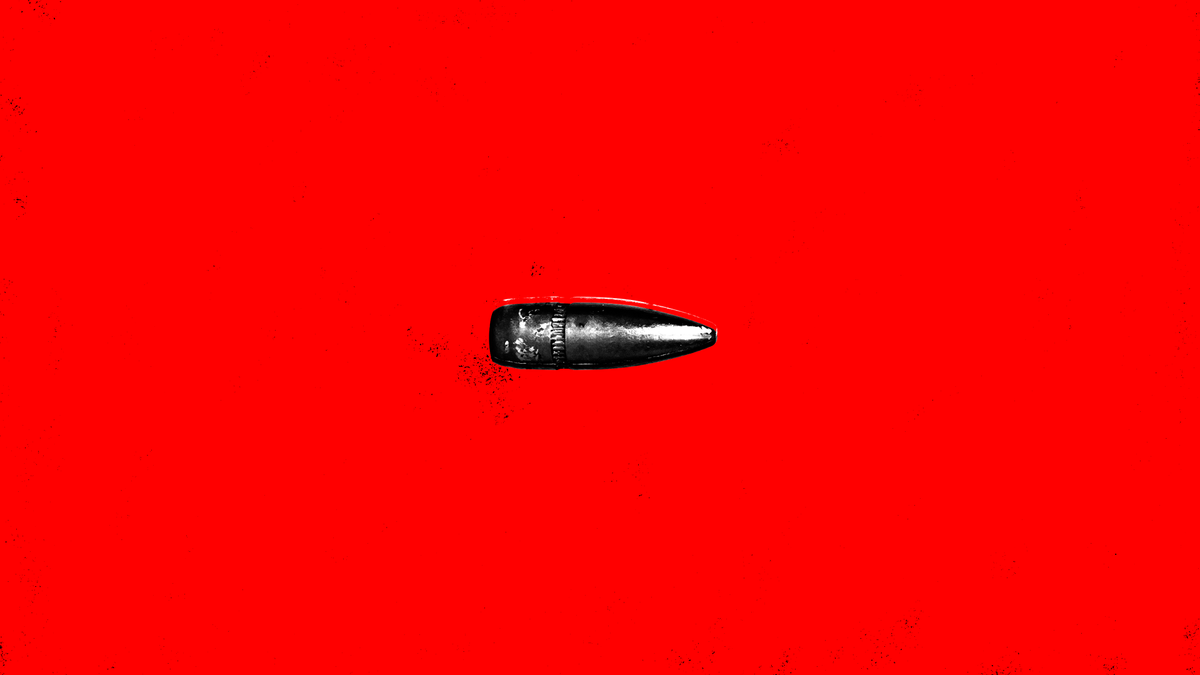The image depicts a meticulous and potentially professionally rendered drawing or illustration of a bullet, centrally positioned against a vibrant, light, juicy red background that carries artistic flair. The bullet itself, likely made of a dark gray or blackened metal such as steel or iron, has a distinctly pointed, cone-shaped tip on the right side, which transitions to a flatter, rectangular left side. This central object, the solitary figure in the image, features a slight glare indicating its metallic texture and shows a ribbed area towards the front. The red background is uniformly bold and bright, accented by subtle distressed areas and hints of black, giving the scene a slightly gritty appearance, much like scattered powder.